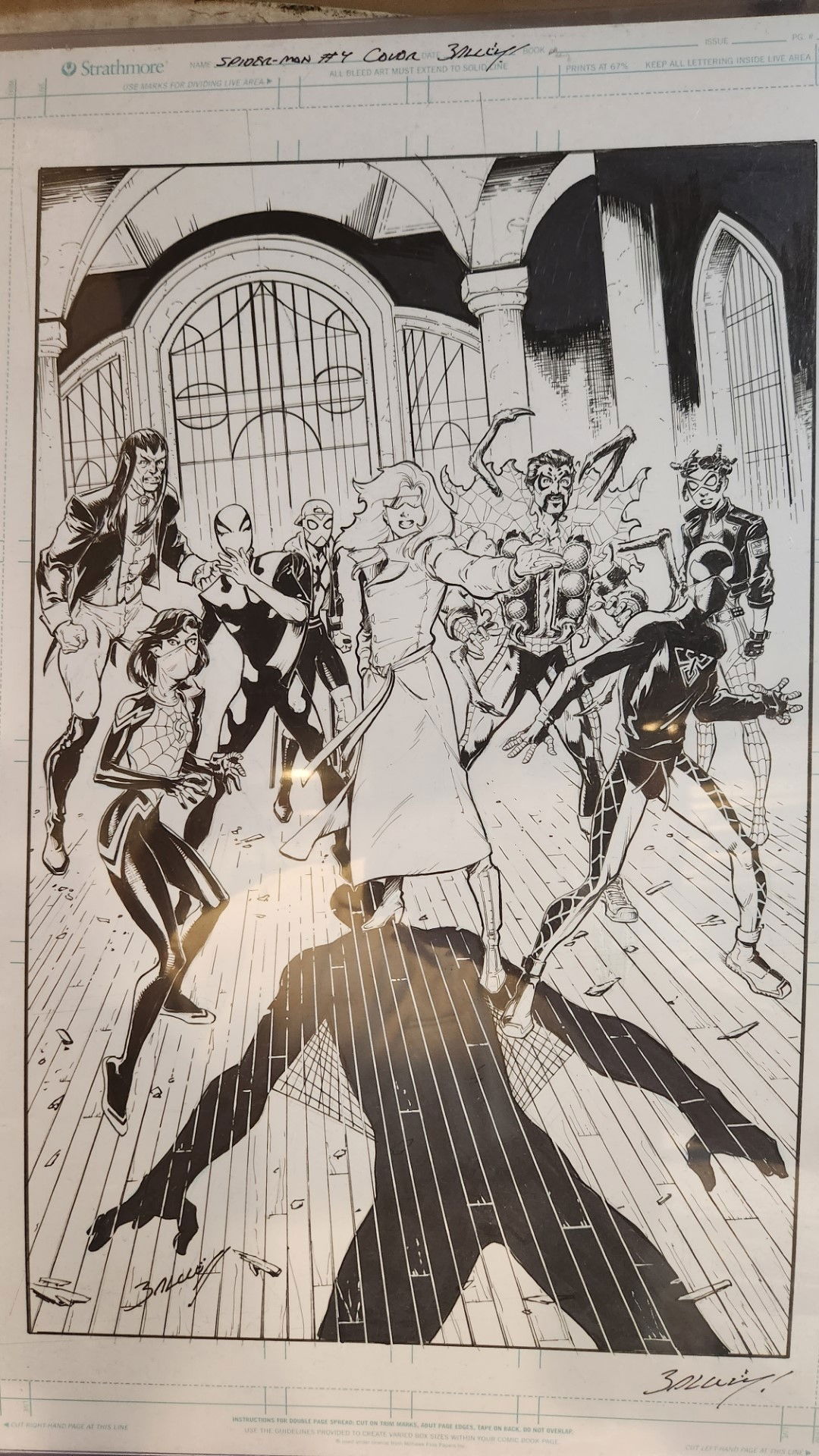This is an intricate black-and-white pen-and-ink drawing, potentially a proof for a comic panel, featuring Spider-Man at the top along with the word "Cobra" and a cursive signature that is hard to decipher. The scene is set in a grand building resembling a church or a place like Grand Central Station, characterized by large arched windows, high ceilings, and pillars. At the center of the composition, a formidable Spider-Man casts a large shadow on the floor, instilling fear among a group of eight characters, who seem to be either superheroes or villains, standing with fearful expressions. The group includes a woman in a white dress and several humanoid figures with insect-like features, including legs and pincers. The detailed shadow and the expressions suggest a confrontational moment, capturing the tension and dramatic atmosphere of the scene.